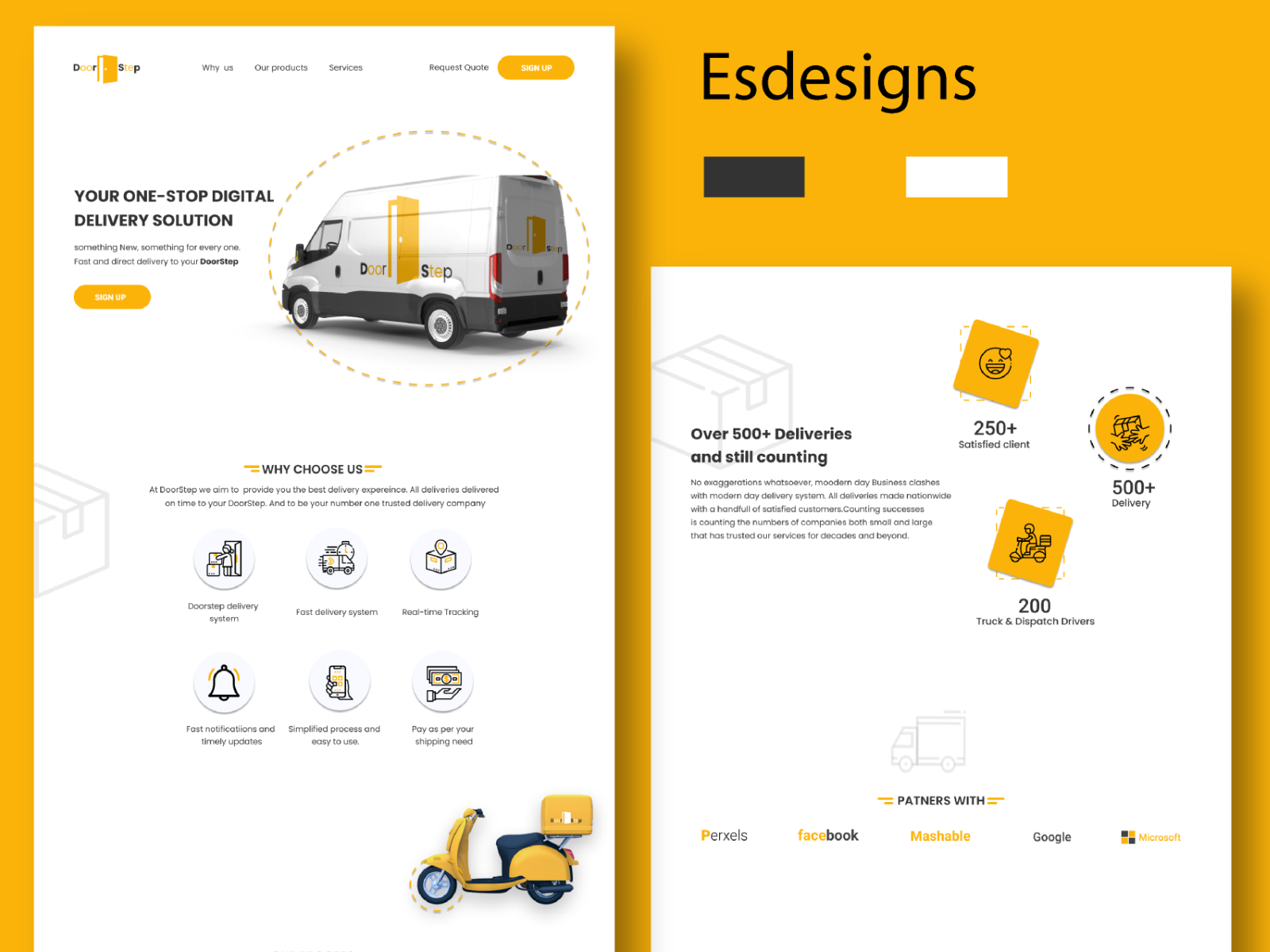**Caption:**

The screenshot features an orange-themed website designed for a digital delivery service. Dominating the left side of the image is a large white rectangular section with a subtle drop shadow, enhancing its prominence. This section, acting as the primary focus, displays the slogan: "Your one-stop digital delivery solution. Something new, something for everyone. Fast and direct delivery to your doorstep." Below this text is an orange oblong button labeled "Sign Up."

Adjacent to this section is a photograph of a white delivery van positioned diagonally with its front facing left. The van is adorned with an illustration of an orange open door, accompanied by the words "Door" on the left side and "Step" on the right side of the vehicle. The same branding is repeated on the back panel of the van. The entire image of the van is accentuated by small lines forming an oval around it.

At the bottom of the left section, a promotional message reads: "Why choose us? At Doorstep, we aim to provide you the best delivery experience. All deliveries are made on time to your doorstep, and we strive to be your number one trusted delivery company." Beneath this message, a list elaborates on the service benefits, including a fast delivery system, real-time tracking, fast notifications and timely updates, a simplified process, and an easy-to-use platform, with payments tailored to shipping needs.

The right side of the screenshot features a shorter white rectangle with a drop shadow. At the top, it displays the text "ES Designs" in capital letters, followed by a logo comprising a black and a white rectangle. Below this, another white section highlights the company's achievements, stating: "Over 500 deliveries and still counting. No exaggerations whatsoever. Modern-day business clashes with a modern-day delivery system. All deliveries made nationwide with a handful of satisfied customers. Counting successes by the number of companies, both small and large, that have trusted our services for decades and beyond."

Additionally, statistics on the left list "250+ satisfied clients, 500+ deliveries, 200 trucks and dispatch drivers," and "Partnerships with PERXELS, Facebook, Mashable, Google, Microsoft."